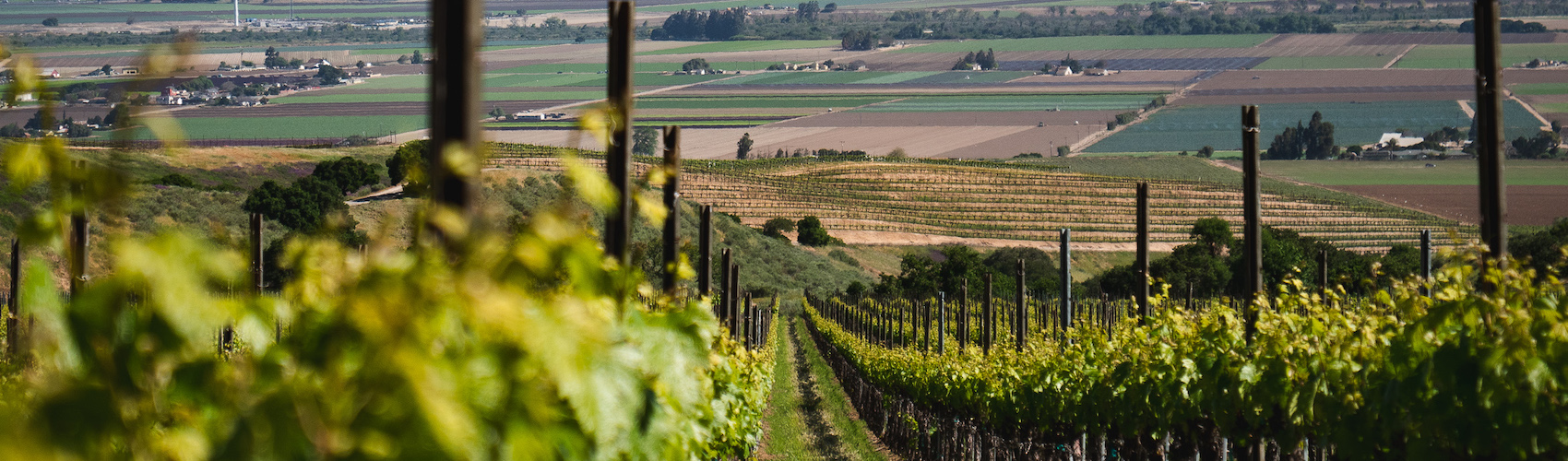This panoramic image, approximately five times wider than it is tall, depicts a vibrant agricultural landscape. In the foreground, we see a well-maintained vineyard with lush, green grapevines climbing trellised posts. The vineyard stretches out in parallel rows from the bottom to the top of the frame, intersected by a pathway or road. The scene captures the meticulous arrangement of the agricultural area, with other distant cultivated fields visible in the mid-ground. These fields display alternating rows of tilled soil and emerging green sprouts, possibly indicating recent planting. Off to the right, a distinctive blue-green field piques curiosity. The backdrop features a row of dark green trees, small houses scattered across the landscape, and a more clustered village to the left. There are also some commercial buildings. The entire scene is bathed in sunlight, enhancing the vibrant greens and earthy tones. There is no visible sky in the image, as the land dominates the view.